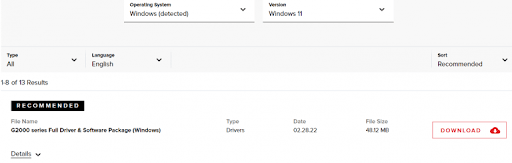The image is a left-to-right horizontal screenshot from a desktop computer running Windows 11. The interface features a mix of gray and white backgrounds. The main section displays the Windows operating system detected and confirmed as version Windows 11, and beneath it are two white boxes on the gray background. 

Located upper left is a drop-down menu labeled "All" for filtering, and the language is set to English with the option to change it using another drop-down arrow. On the far right side, there’s a "Sort" option, currently set to "Recommended" with an arrow to adjust the sort criteria. The interface indicates it’s showing "1 to 8 of 13 results," and a horizontal line separates this section from the content below.

The highlighted content shows a black box with uppercase white letters reading "RECOMMENDED." Below is a detailed file description: "G2000 series full driver and software package (Windows)." The file type is labeled "Drivers," with a date of "2/28/22," and a file size of "48.2 MB." To the right, a red "Download" button is prominently displayed. On the left side, there is an underlined "Details" option with a small arrow for additional information.